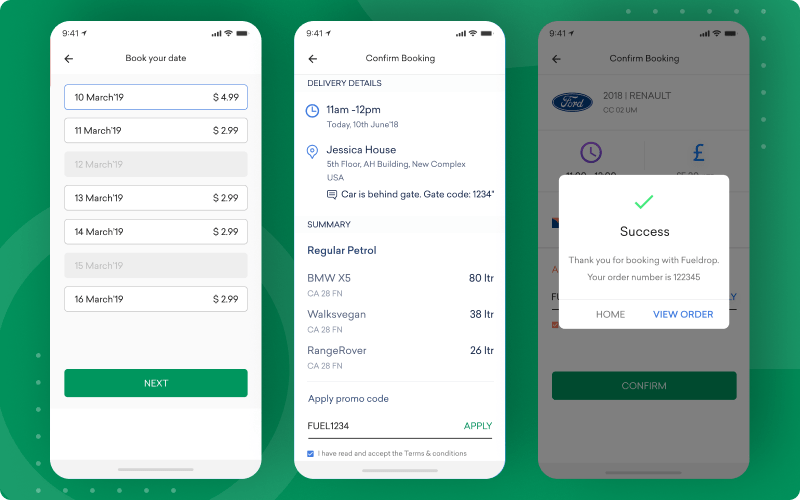The image features a large, greenish rectangle as the background, embellished with some subtle design elements. Superimposed on this backdrop are three smartphone screens aligned side by side, effectively demonstrating a step-by-step process for booking and confirming a car order.

The first screen displays a date selection interface. The user is prompted to "Book your date" with options starting from March 10, 2019, to March 11, 2019. The first date (March 10) lists a price of $4.99, while subsequent dates such as March 11, 13, 14, and 16, each show a price of $2.99.

The second screen moves on to delivery details, specifying a delivery window from 11 AM to 12 PM at "Jessica House, 5th floor, A.H. Building, New Complex, USA." Additional notes indicate that the car will be behind a gate with the access code 1234. A summary section lists available car types (BMW, Volkswagen, Range Rover) and their respective fuel requirements, specifying regular petrol and the number of liters involved.

The third screen confirms the booking with the text "Success" and a mention of "Ford Renault" in the background, providing an indication that the order process has been completed.

The overall sequence suggests a detailed and secure process for ordering a car, from selecting dates and delivery specifics to final confirmation.